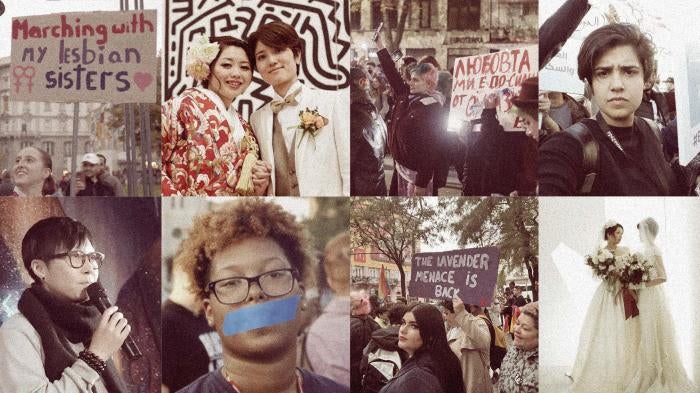This image is a collage of eight square photos arranged in a four by two layout, each depicting moments related to lesbians and women. The top left photo shows a woman holding a sign that says "Marching with my lesbian sisters," amidst a group of people marching. To the right, two Asian women are captured in a tender moment, possibly on their wedding day, with one in a kimono and the other in a white suit. Next, another protest scene includes women holding up a sign in Russian. The fourth photo on the top row features a woman with short hair and a somber expression, wearing a black shirt, with protest signs in the background.

On the bottom row, the first photo depicts a person with black hair and glasses holding a microphone, perhaps about to speak. This is followed by an image of a woman with blue tape over her mouth, wearing glasses. The third photo shows people holding a sign that reads "The Lavender Menace is Back," possibly at a protest or march. The final photo captures two women in elegant wedding gowns, holding bouquets and looking at each other affectionately.